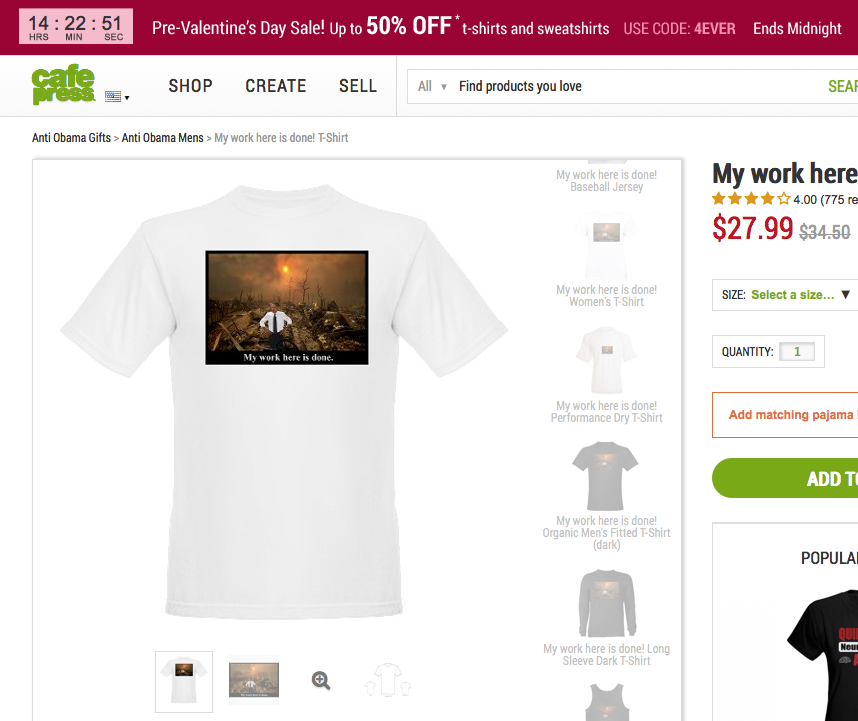This image showcases a screenshot taken from a desktop or laptop computer, displaying the homepage of the CafePress website. CafePress is an online platform that allows users to order custom-made clothing, coffee mugs, and other personalized items. 

In the top left corner of the site, a countdown timer is prominently displayed on a red banner background, indicating 14 hours, 22 minutes, and 51 seconds remaining until the end of a sale. To the right of the timer, white text on the red banner announces a "Pre-Valentine's Day Sale" with discounts of up to 50% off on t-shirts and sweatshirts, urging customers to use the code "FOREVER" before the offer ends at midnight.

Directly below the red banner, a white header features the CafePress logo in a green lowercase font, accompanied by a language and region dropdown menu on the right. Adjacent to this are navigation buttons labeled "Shop," "Create," and "Sell," alongside a product search bar.

The content beneath this header includes a category listing titled "Anti-Obama Gifts" with a focus on "Anti-Obama Men's" t-shirts. The highlighted product is a plain white t-shirt bearing the name "My Work Here is Done T-Shirt," priced at $27.99, reduced from its original price of $34.50. The t-shirt features a photograph of former President Barack Obama standing amidst the rubble of what appears to be a devastated town, set against a dark, somber sky. Positioned below the image is the caption, "My work here is done." Additional varieties of the same t-shirt are visible on the side of the product listing.